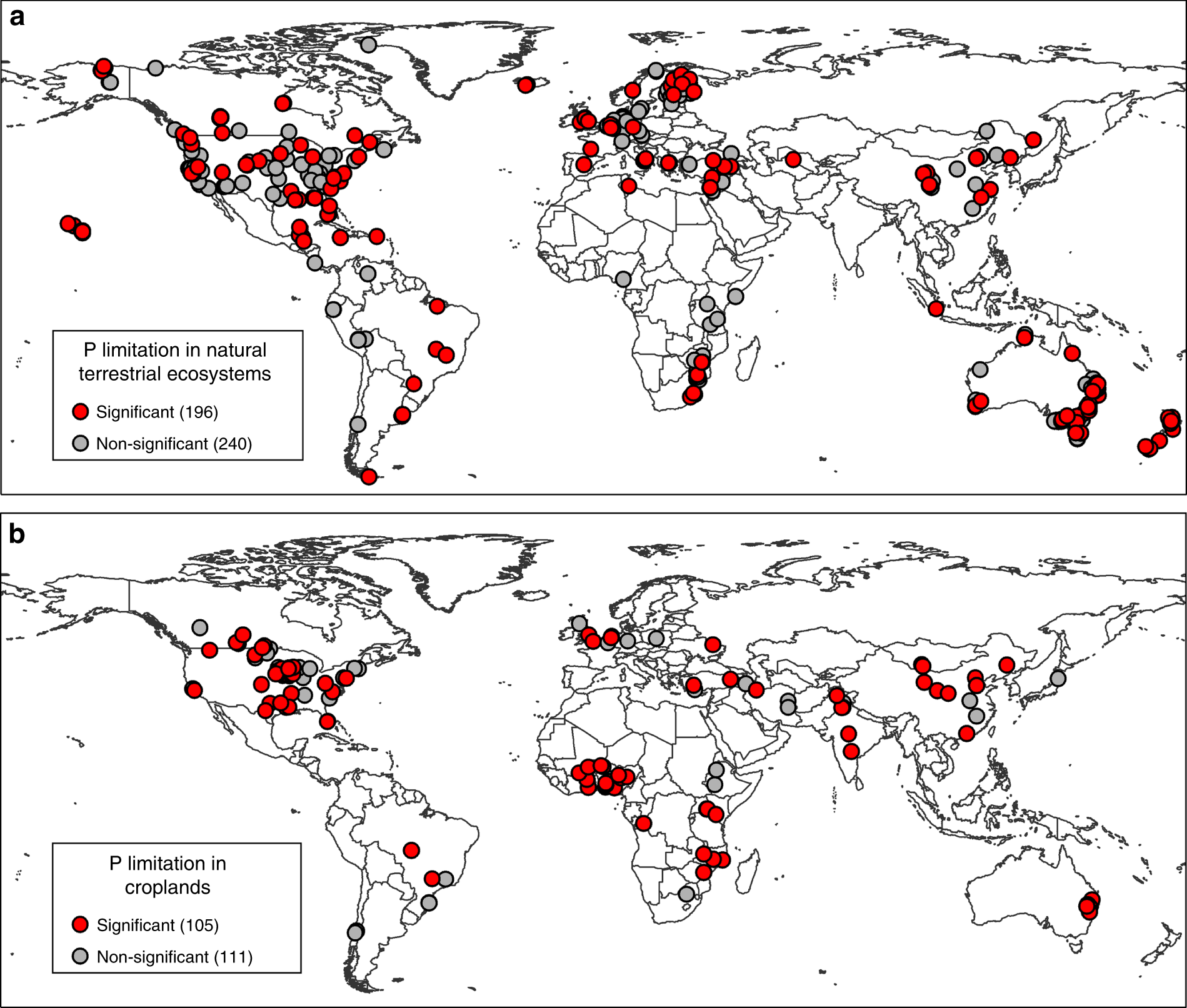This image showcases two detailed world maps, stacked vertically, each portraying P limitation data. Both maps share a monochromatic base with black contour lines against a white background, accented with numerous red and grey dots indicating significant and non-significant points respectively.

The map on top is titled "P Limitation in Natural Terrestrial Ecosystems." It features a legend in the bottom left corner, specifying that red dots (196 in total) denote significant P limitation, while grey dots (240 in total) represent non-significant P limitation. A dense distribution of red dots can be observed along the east and west coasts, as well as the northwest and midwest regions of the United States. Brazil and Latin America also exhibit many red dots, with some grey dots appearing along Brazil's west coast. Africa has a sparse distribution, with red dots concentrated near the southern tip and a few in northern Africa. Europe displays a substantial cluster of red dots, whereas China has about eight red dots. Notably, Russia is devoid of any dots, and Australia shows red dots primarily along its east coast.

The lower map is titled "P Limitation in Croplands," with a corresponding legend indicating red dots (106 in total) as significant and grey dots (111 in total) as non-significant. Here, the red dots are again prevalent across the United States, though this map shows a higher concentration of red dots in West Africa and the southern tip of Africa. India has four red dots, Europe around six, China about six, while Russia remains dot-free. Australia has one or two red dots with very few grey dots.

These maps collectively illustrate the geographical distribution and density of phosphorus limitation in both natural terrestrial ecosystems and croplands, with a focus on red dots representing significant data points across various continents.